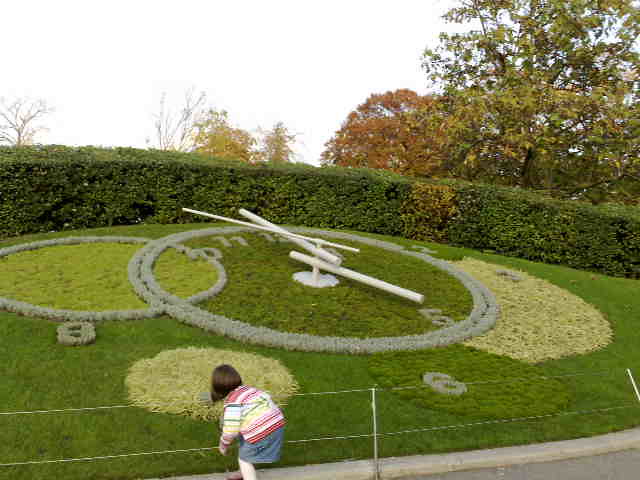This daytime photograph captures a detailed ornamental grass sculpture designed as a clock face embedded into a grassy slope. The clock, featuring large tubular white hands including a second hand, displays a time of five o'clock. Surrounding the clock are numbers formed within circular hedges and edging plants, with notable digits like 10, 11, 12 at the top, 5 within the circle, and 6 at the bottom. A thin cable railing runs along the sidewalk in front of this intricate design, demarcating the sculpture from the observer's path.

In the foreground, a little girl dressed in a denim skirt and striped sweater, with shoulder-length hair, is bent over near the railing, possibly examining the fence or attempting to look beyond it. At the top of the slope, the clock is crowned by an arched shrubbery. The background complements the scene with trees adorned in autumn colors, adding to the picturesque environment of the garden-like setting.